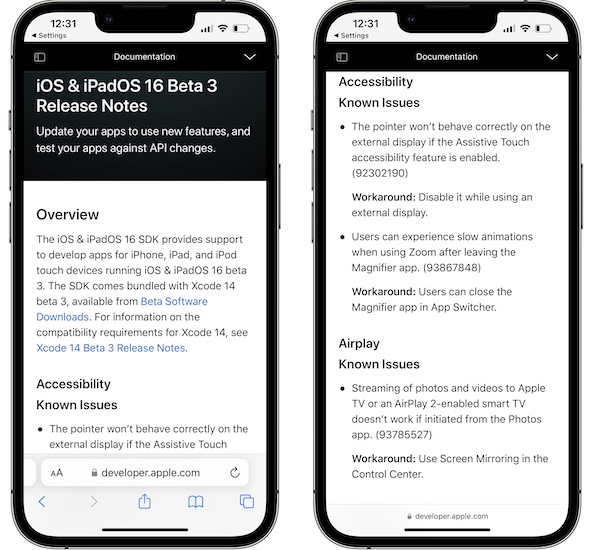This image features two smartphones positioned side-by-side, each displaying text content on their screens. Both phones exhibit a status bar at the top, showing a time of 12:31 with a nearly depleted battery icon on the right. The phones have a white background with black text.

The phone on the left displays a document titled "iOS and iPadOS 16 Beta 3 Release Notes." The text encourages users to update their apps to leverage new features and test them against API changes. This section is set against a black background. Beneath this, the document presents an "Overview" heading followed by an "Accessibility" section. The visual layout continues with a "Known Issues" subsection, detailing various known issues and linking to developer resources at the bottom of the screen, indicated by "developer.apple.com."

The phone on the right appears to continue from the first phone's document, proceeding with the "Accessibility" section. It includes a "Known Issues" segment that lists two bullet points, each describing specific issues and providing workarounds. Following this, an "AirPlay" section outlines another set of known issues, presenting one bullet point with an accompanying workaround option.